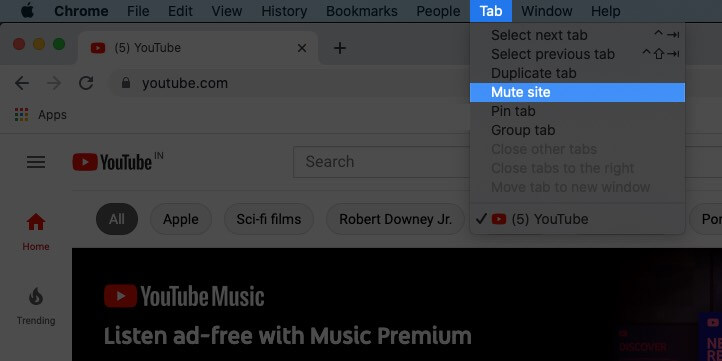The image depicts a web page with a dark gray overlay, likely indicating an incognito or private browsing mode. At the very top, a browser menu bar displays the following options: 'Chrome,' 'File,' 'Edit,' 'View,' 'History,' 'Bookmarks,' 'People,' 'Tab' (which is highlighted), 'Window,' and 'Help.' Below this, the open tab reads "5 YouTube," accompanied by the YouTube icon on the left side.

On the YouTube page, the upper left corner features the menu icon represented by three horizontal lines, followed by the word 'YouTube' next to the familiar logo. A white search bar is prominently displayed. Below the search bar, several buttons are visible, with 'All' being highlighted in dark with white text, indicating it is currently selected. Additional buttons to the right read: 'Apple,' 'Sci-Fi Films,' and 'Robert Downey Jr.'

Along the left side of the YouTube interface, prominent icons and labels include 'Home' with a red home icon beside it, and 'Trending' accompanied by a fire icon above it, indicating popular or trending content on the platform. The overall layout is clear and focused on content navigation within YouTube.